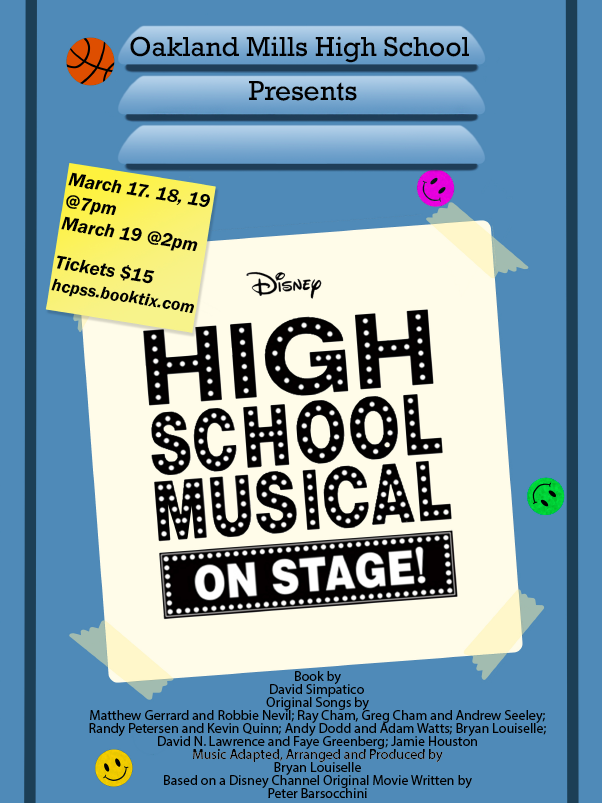The image is a flyer, designed to look like the front of a school locker, advertising a high school musical put on by Oakland Mills High School. Against a blue background, the top section mimics locker vents and reads "Oakland Mills High School presents." Below, a white paper-like section, as though taped to the locker, announces "Disney's High School Musical on stage" in large uppercase black text with tiny lights, giving it a marquee effect. The flyer also features a prominent yellow sticky note displaying information about showtimes: March 17th, 18th, and 19th at 7 p.m. and an additional matinee on March 19th at 2 p.m. Tickets are priced at $15 and can be purchased via hcpss.booktix.com. The locker door is adorned with various stickers, including happy faces and a basketball, adding to the school-themed decor. At the bottom, it lists credits for the show's book and music, attributing various original songs and arrangements to a team of composers, highlighting contributions by David Simpatico, Matthew Gerrard, Robbie Nevil, among others, and emphasizing its origin as a Disney Channel original movie.